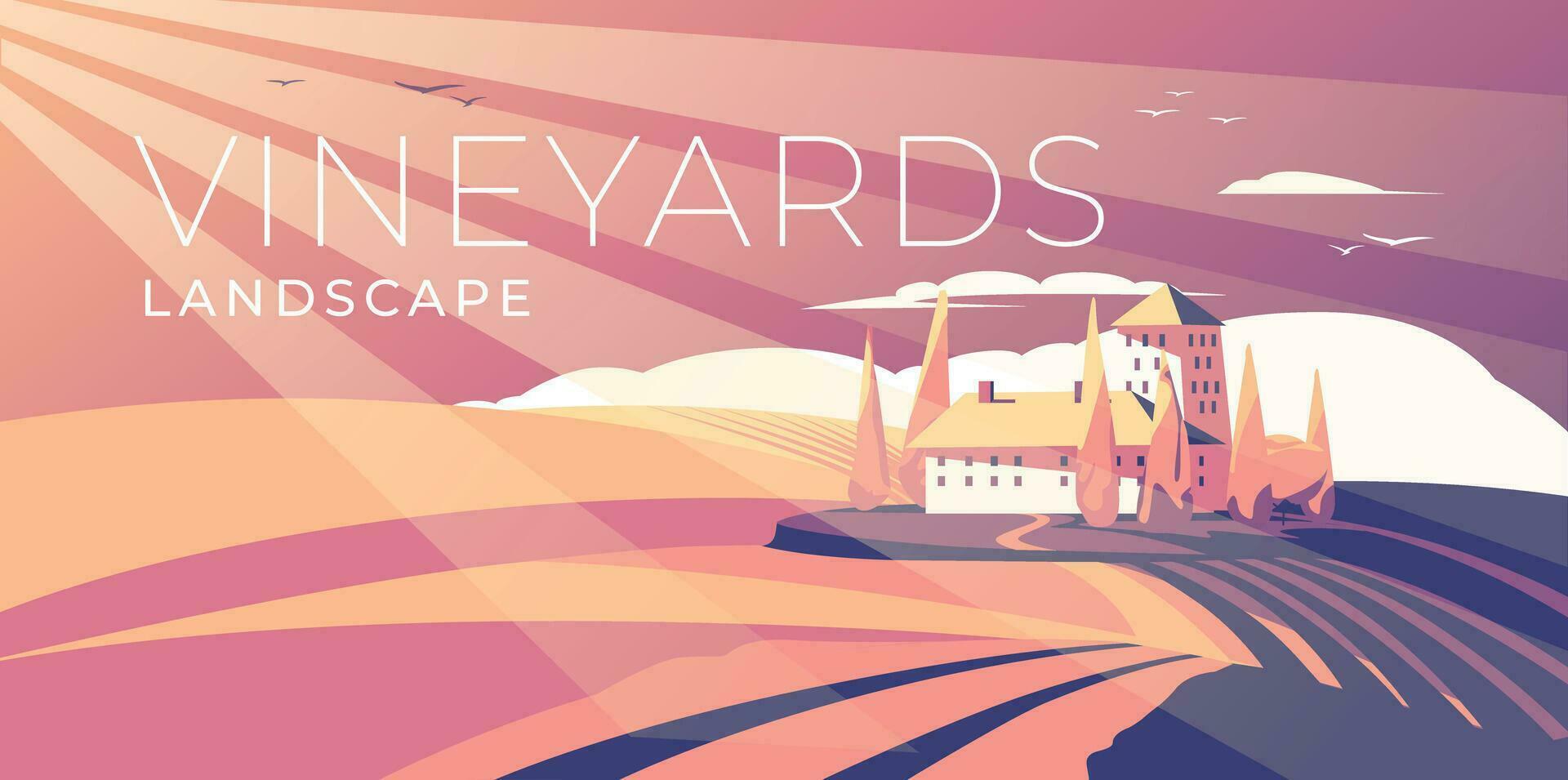The image is a colorfully artistic digital render of a scenic vineyard landscape. Dominating the scene is a stylized, large mansion situated amidst expansive fields and trees. The mansion features a two-story rectangular section with a peaked roof, two chimneys, and ten windows on one face. Behind this structure rises a taller, narrower tower-like building, also adorned with numerous windows and a peaked roof.

The sky transitions from an orange-tinged hue on the left to a rich purple on the right, embellished with stylized white clouds. A brilliant sunset in the upper left corner sends four distinct rays of light, in a light yellowish color, diagonally across the sky towards the lower right corner. The fields, rendered in varying shades of orange and dark purple striping, stretch out in front of the house, guiding the viewer’s eye with a road that leads directly to the mansion. Orange-toned trees dot the landscape, harmonizing with the warm palette of the scene.

In the foreground, elegant white lettering spells out "Vineyards Landscape" in the center, adding to the artistic character of the illustration. The simplicity of lines and the blend of uniform colors, from yellow and pink to black, convey a harmonious yet striking visual experience.